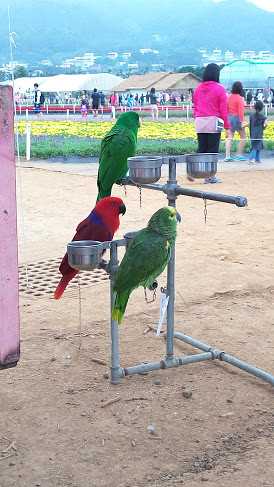This image depicts a vibrant scene where three parrots—two green and one red and blue—are perched on a stand within an outdoor setting that could be a zoo, farm, or festival. The green parrot nearest to the viewer displays a hint of yellow on its face, while all three birds are tethered to their perch, seeming to observe the bustling activity around them. Surrounding the birds' stand, which houses tins of bird food, is a dirt pathway that transitions into a sidewalk.

In the middle of the frame, a lush bed of yellow flowers adds a splash of color. The background reveals a lively scene with numerous people walking, including what appears to be a mother and her daughter, and another lone woman nearby. Beyond this, there is a collection of makeshift tents and market-style structures, indicative of a festival or local bazaar, with a cityscape stretching across hills in the distance. Adding to the scene’s picturesque quality are mountains rising against the horizon, further enhancing the image's blend of natural beauty and human activity.